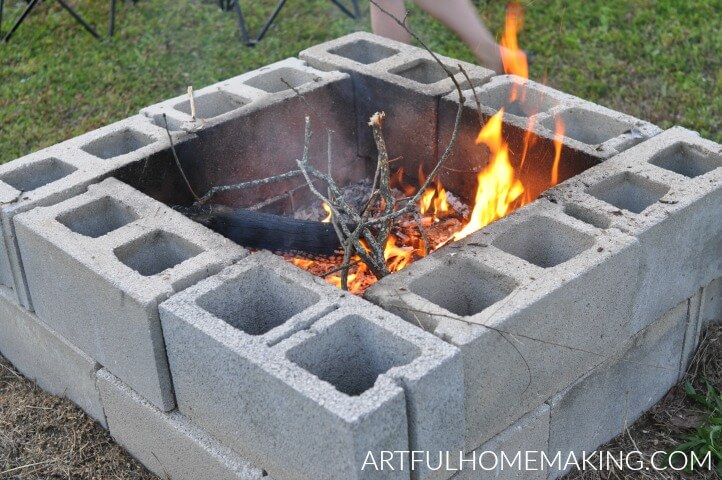This outdoor image showcases a makeshift fire pit constructed from two layers of grey cinder blocks arranged to form a square. The interior of the cinder blocks is visibly blackened from soot, evidence of previous fires. Inside the fire pit, there are dead branches, bramble, and leaves, with flames leaping from their burning centers. The fire pit is situated on a low rising patch of green grass. In the background, slightly blurry, are the legs of a person, presumably seated in lawn furniture or camping chairs, adding to the casual outdoor setting. Additionally, a URL reading "artfulhomemaking.com" is visible in the bottom right corner of the photograph.